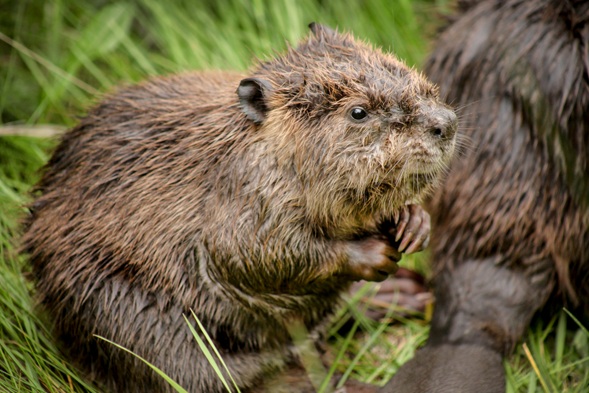This close-up image features a young beaver prominently positioned in the center, occupying most of the middle of the frame. The baby beaver's fur is a mix of brown hues with hints of lighter tan and appears slightly wet, suggesting recent activity in water. Its beady black eye is focused to the right, and its tiny white whiskers add a delicate touch to its face. The beaver is nestled in green grass, approximately 5-6 inches tall, with its two front paws clasped together, giving a detailed view of its face, legs, and tail. On the right side, the mother beaver is visible, though somewhat blurry, showing only her hindquarters and part of her distinctive beaver tail near the bottom right corner, contributing to the sense of depth and setting.